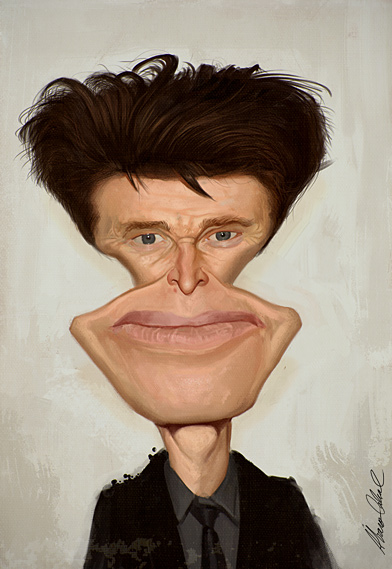This is a digitally created, cartoon-style illustration of a man characterized by its highly distorted features. The man's face exhibits triangular-shaped eyes and cheek areas, a diamond-shaped mouth and chin, contributing to a visually intriguing and bizarre appearance. His neck is elongated, while his body, clad in a black suit with a grey collared shirt and a black tie, remains quite normal. The depiction is focused on his upper body—primarily a shoulder headshot—positioned so that he is looking straight forward. The background is a simple off-white color with grey shading in the corners. Additionally, there is a black signature on the right side of the illustration, oriented upwards. Notable colors in the piece include tan, light pink, dark gray, black, off-white, grey, brown, and dark blue for the eyes.